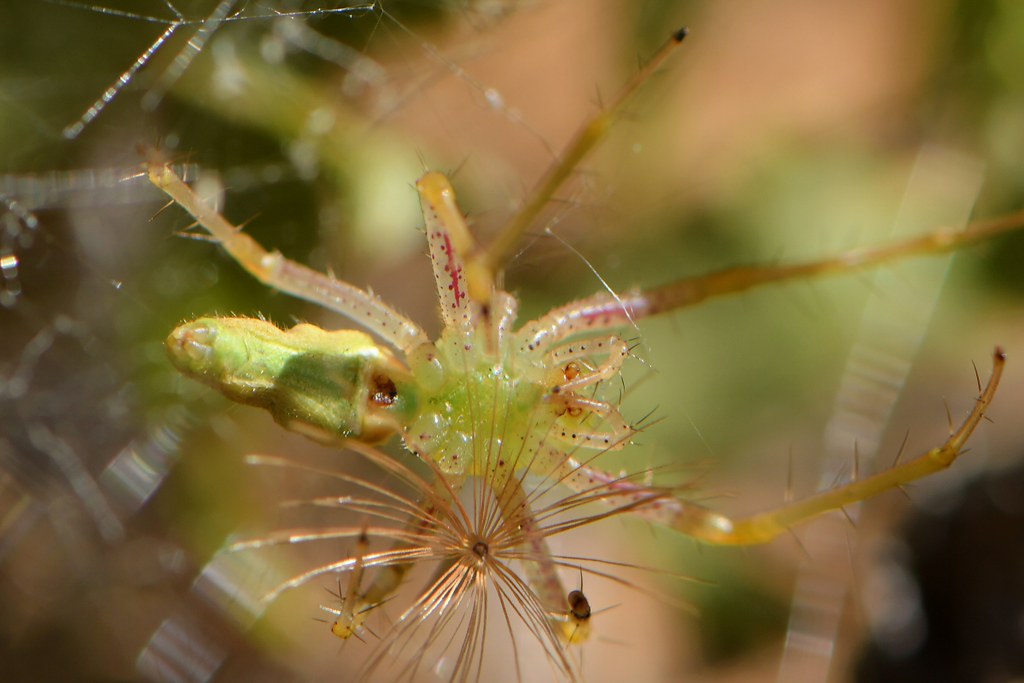In this detailed image, we see a spider with a light green body adorned with subtle yellow highlights and translucent areas. Its almost clear legs exhibit magenta streaks and black spots near the joints, creating an intricate appearance. The spider is set against a blurred background where sections of green and light purple are faintly visible. Distinct strands of webbing can be seen, hinting at the spider's environment. Additionally, there is a small flower with long, beige, eyelash-like stems that appears to be attached to the web, along with a couple of tiny bugs that the spider may be feeding on. The combination of detailed close-up focus on the spider and the more indistinct background elements contributes to a composition that emphasizes the delicate yet striking features of the spider and its immediate surroundings.